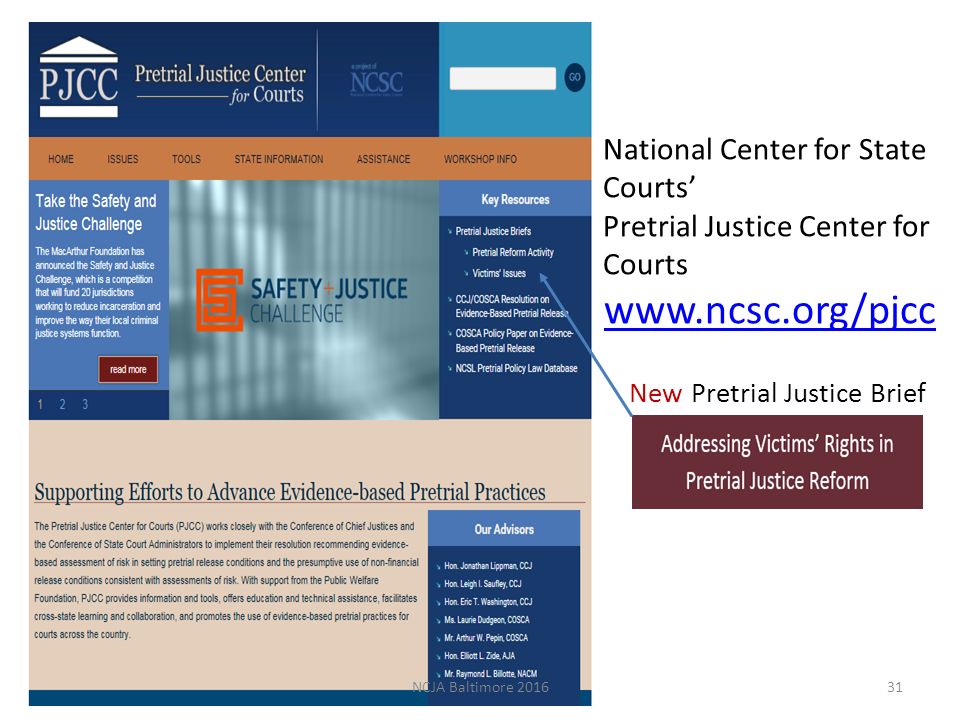The image displays a header area with a dark blue background transitioning to light blue on the top right corner. On the left side of the header, the acronym "PJCC" is prominently displayed, standing for the "Pre-Child Justice Center for Courts," alongside the acronym "NCSC." Below the header, there is a brown navigation menu with clickable options labeled: Home, Issues, Tools, State Information, Assistance, and Workshop Info.

To the left below the navigation menu, a light purple-colored box features the text "Take the Safety and Justice Challenge." Adjacent to this box, on the right, there's an image depicting jail bars, symbolizing a jail cell, with the caption "Safety and Justice Challenge."

Beneath these elements, a light pink-colored box contains the call-to-action "Support an Effort to Advance Evidence-Based Pre-Trial Practices." Further down, text explains that the Pre-Child Justice Center for Courts (PJCC) collaborates closely with the Conference of Chief Justices and the Conference of State Court Administrators. This partnership is aimed at implementing resolutions that endorse the evaluation of risk in pre-trial release conditions using evidence-based assessments, and advocate for the presumptive use of non-financial release conditions that align with these assessments.